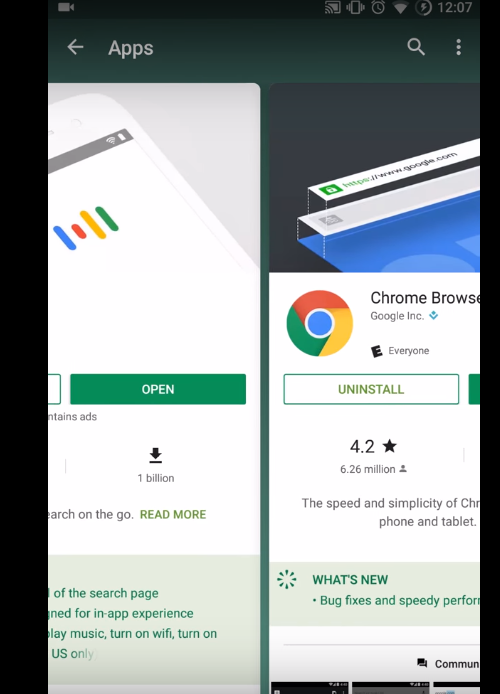This screenshot depicts a section of a web page related to the Google Chrome app. At the top of the image, there is a navigation bar featuring a left-pointing arrow labeled "Apps," a search icon, and a three-dot menu icon for additional options.

The upper part of the screenshot includes an image that appears to be a collage of two pages. On the left, we observe the familiar Google Chrome colors, accompanied by a green rectangular button with the white text "Open." Directly below this button, there is a downward-pointing arrow with a line, followed by text that is partially obscured but appears to begin with "1 billion." Under this, the phrase "Search on the go" and "Read more" are visible.

Next to this section, the Google Chrome logo—a circular emblem featuring red, yellow, green, and blue segments—is prominently displayed. To the right of the logo, the text reads "Chrome Browser Google INC," denoting the application's developer. Below the name, a rating of "E for Everyone" is shown, along with a white rectangular button bearing the green text "Uninstall." Underneath this button, the app's rating is indicated as "4.2 stars" from approximately "6.2 million" reviews, although the exact number is somewhat difficult to discern due to its small size. Accompanying this information is a brief description: "The speed and simplicity of Chrome, for phone and tablet."

At the bottom of the partially visible page, a rectangular banner announces recent updates with the text "What's new: Bug fixes and speed performance improvements."

Note: Some elements of the text are partially obscured and recognized based on context.